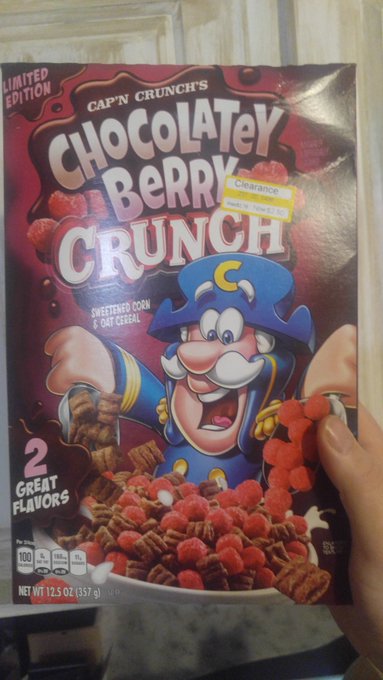The photograph, though poorly lit and likely taken in a home, features a box of Cap'n Crunch's Chocolaty Berry Crunch cereal. The brown-background box has "Limited Edition" noted in the upper left corner, alongside a "clearance" sticker in the upper right. Prominently in the center, the cereal name is displayed over a splash of chocolate with berries peeking behind the text. At the bottom center, there's Captain Crunch, depicted as an admiral wearing a blue uniform and a hat with a yellow "C." He has a white mustache and a pale complexion, holding a spoonful of the cereal consisting of chocolate rectangular biscuits and red berries. Below him, a white bowl filled with the cereal is visible, with a woman's hand holding the box from the bottom right corner. In the background, a partially visible, dirty white door with grayish marks can be seen, adding to the homey setting of the image.